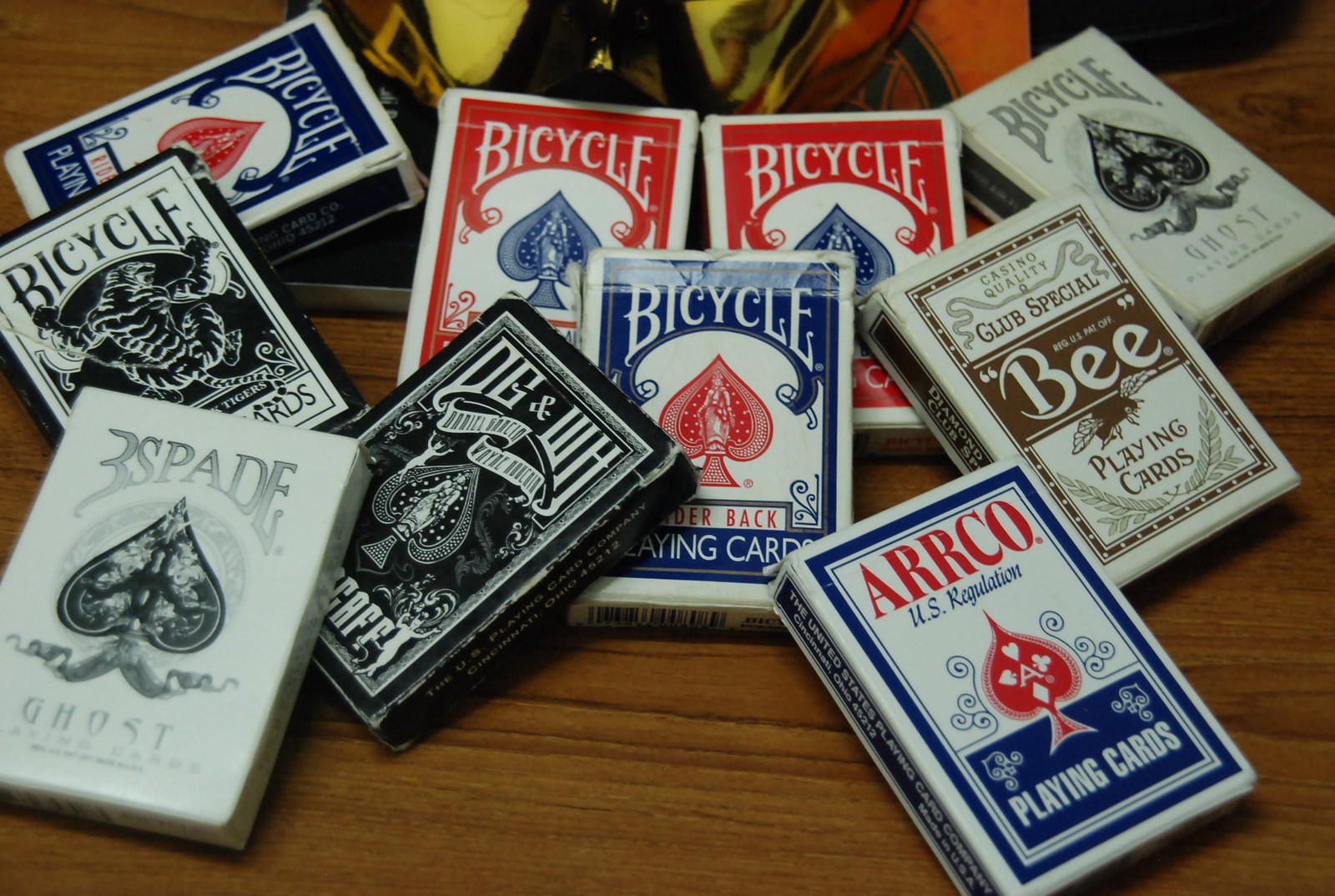The image showcases an assortment of playing card boxes organized haphazardly on a brown wooden table with various objects in the background. Featured prominently are five different Bicycle brand decks: two in red and white with blue spades, two in blue and white with red spades, and one in black and white alongside another in white and gray. Alongside these are two packs of Three Spade cards which are black and white with gray lettering, and a single Arco deck in white and blue with red text. Completing the collection is a pack of Club Special "B" cards, distinguished by their brown and white design. In total, there are ten packs of cards, each adding to the diverse array of color schemes and brands displayed.